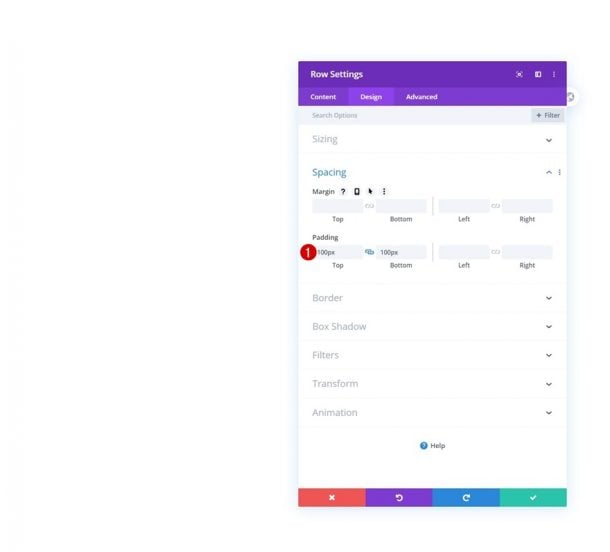In this screenshot, we are presented with a user interface showcasing a website or application customization menu. At the top, a purple header displays in bold white text the title "Settings" located in the upper-left corner. Just below the header, there is a menu bar featuring three action buttons labeled "Content," "Design," and "Advanced."

Moving further down, a search option is visible, followed by a section starting with the option "Sizing" written in light gray text accompanied by a pull-down arrow on the right. Underneath, the word "Spacing" appears in blue text. Directly below "Spacing," we see the term "Margin" in small black text with a question mark icon next to it, likely providing more information or help. Followed by this, the word "Padding" is highlighted in bold text.

On the left side of the interface, there are additional options listed in light gray text, each with a pull-down arrow to the right: "Border," "Box Shadow," "Filters," "Transform," and "Animation."

In the center of the lower part of the menu, the word "Help" is visible in small text, accompanied by a small blue circle housing a white question mark to the left, suggesting assistance or further information is available here.